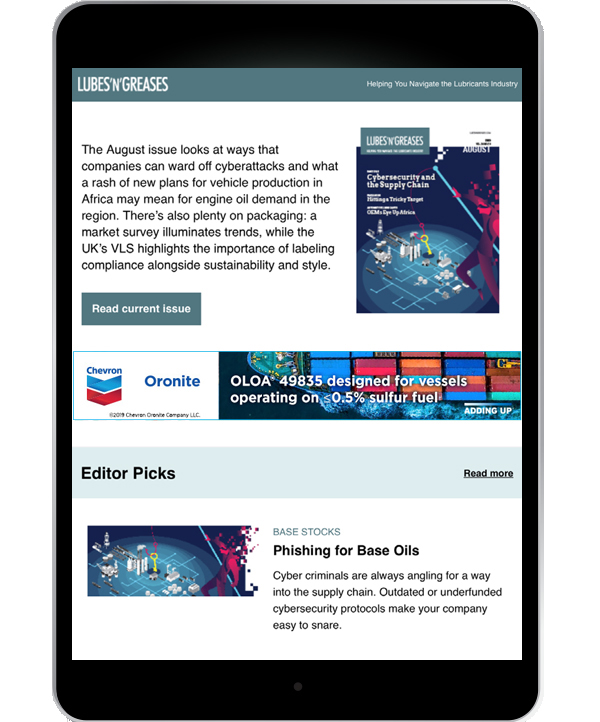The informational area features a black outline with a green rectangle to the left, inside of which "Lubes & Greases" is written in uppercase letters. Below this, in black text, the caption details the August issue's focus. It explores strategies that companies can use to prevent cyber attacks, examines the implications of new vehicle production plans in Africa on regional engine oil demand, and delves into packaging trends. A market survey sheds light on these trends, with input from the UK's VLS stressing the importance of competent labeling, sustainability, and style.

Below the main text, another green rectangle prompts readers to "Read Current Issue." Beneath this prompt, the word "Chevron" is displayed with banners in blue and red underneath. Further to the right, the word "Oronite," spelled O-R-O-N-I-T-E, appears. To the right of "Oronite," uppercase letters spell out "OLOA 49835," indicating a product designed for vessels operating on 0.5% sulfur fuel. Below this text, a blue rectangle highlights "Editor's Pick," and to its right, another section discusses "Base Stocks," encouraging readers to delve into the subject of fishing for base oils.